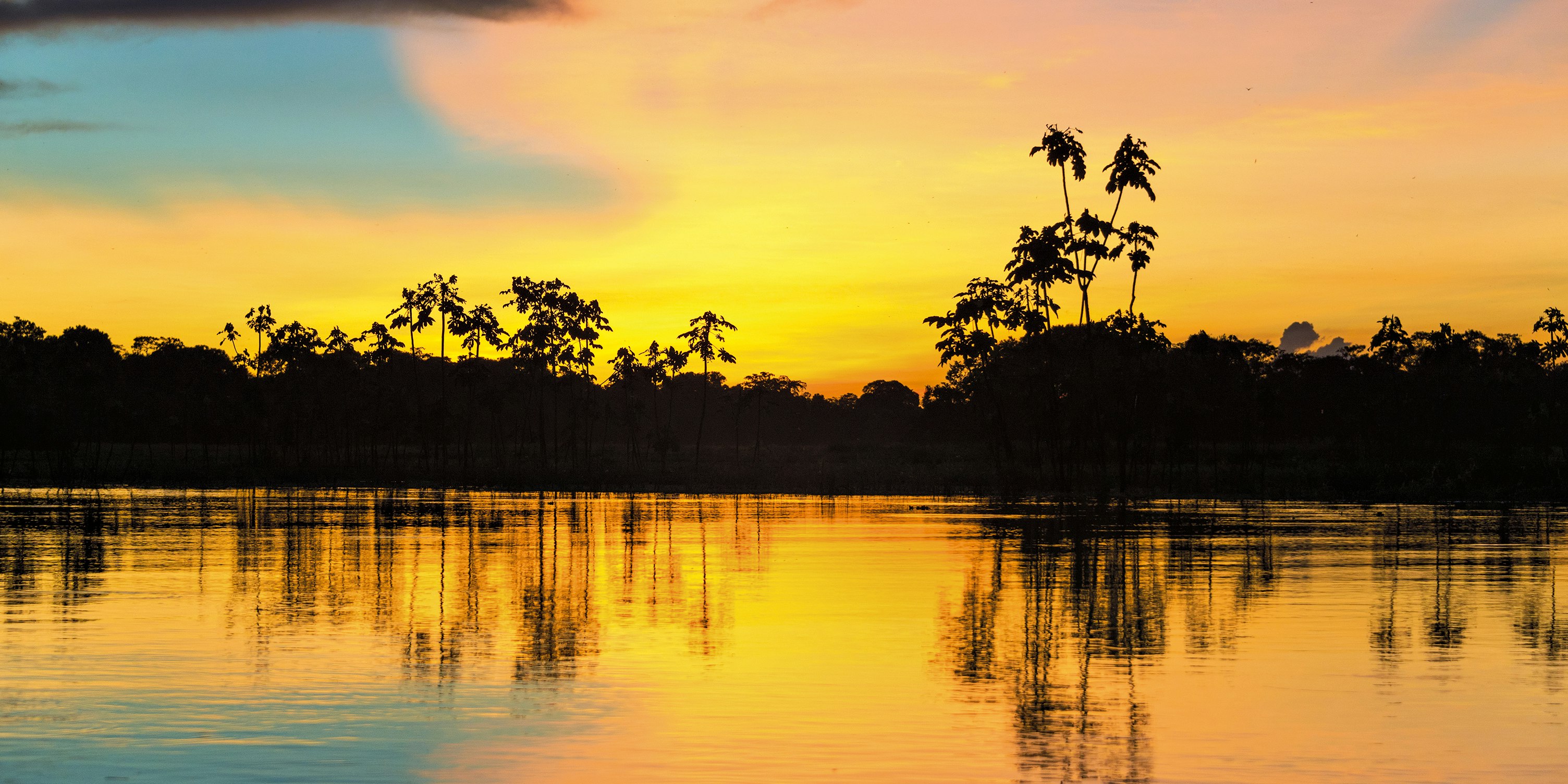The image captures a serene outdoor scene, likely taken during sunset or sunrise, as the sky is adorned with beautiful hues of blue, pink, yellow, and orange. The horizon showcases a dense forest with tall, large trees, their silhouettes creating a striking contrast against the colorful sky. In the top left corner of the sky, there is a remnant of blue, perhaps hinting at the fading daylight. The expansive body of water beneath mirrors this vibrant palette, showing reflections of the oranges, yellows, light pinks, and bits of blue from the sky. The water appears calm and still, enhancing the tranquility of the scene, and it stretches horizontally from the far left to the far right, fully encompassing the reflected silhouettes of the lush vegetation. Overall, it’s a picturesque sunset or sunrise over a vast, serene lake, surrounded by an abundance of trees, capturing nature's beauty in a harmonious blend of light and reflection.